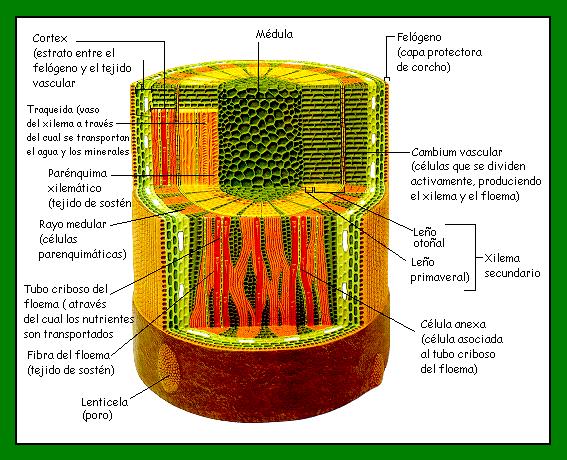The image is a detailed, animated diagram of a biological structure, likely derived from a biology textbook and focusing on a cylindrical cross-section of a vein leading to the brain. The center of the diagram highlights the medulla, a spongy and complex area, indicating its association with brain anatomy. The intricate interior is visible through flat, cut-out segments showcasing multicolored layers and what appears to be biomaterial resembling lava flow. Text labels, written in Spanish, are connected by line segments to various parts of the structure, including mentions of the medulla and cortex. The diagram features vivid, animated coloration with greens and yellows, enhancing its interactive and educational nature.